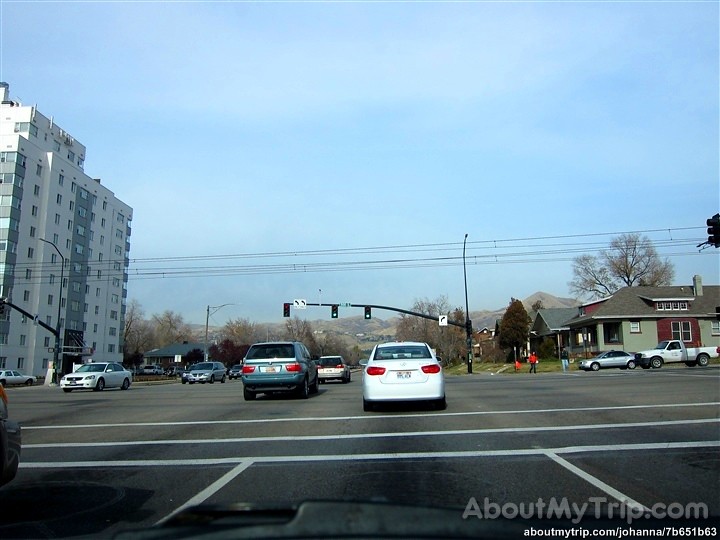This color photograph captures a daytime street scene viewed from inside a car through the windshield. In the foreground, the car's dashboard is visible, providing a sense of being inside the vehicle. Ahead, the street extends into the distance, featuring a crosswalk marked by two solid white lines. Beyond the crosswalk, a white car is directly in front, with a blue SUV positioned to its left. The street comprises two lanes in each direction and is paved with asphalt with clearly marked white lines.

A green traffic light hangs overhead from a pole, indicating go. The sky above is light blue, suggesting clear weather. On the upper left side of the image, a tall white and gray building, resembling an apartment complex, stands prominently, adorned with numerous small square windows. To the right, a residential house with light green siding and a gray roof can be seen. Electrical power lines span the width of the photograph, running horizontally across the scene. This detailed image encapsulates a typical urban intersection, poised for the next move forward.